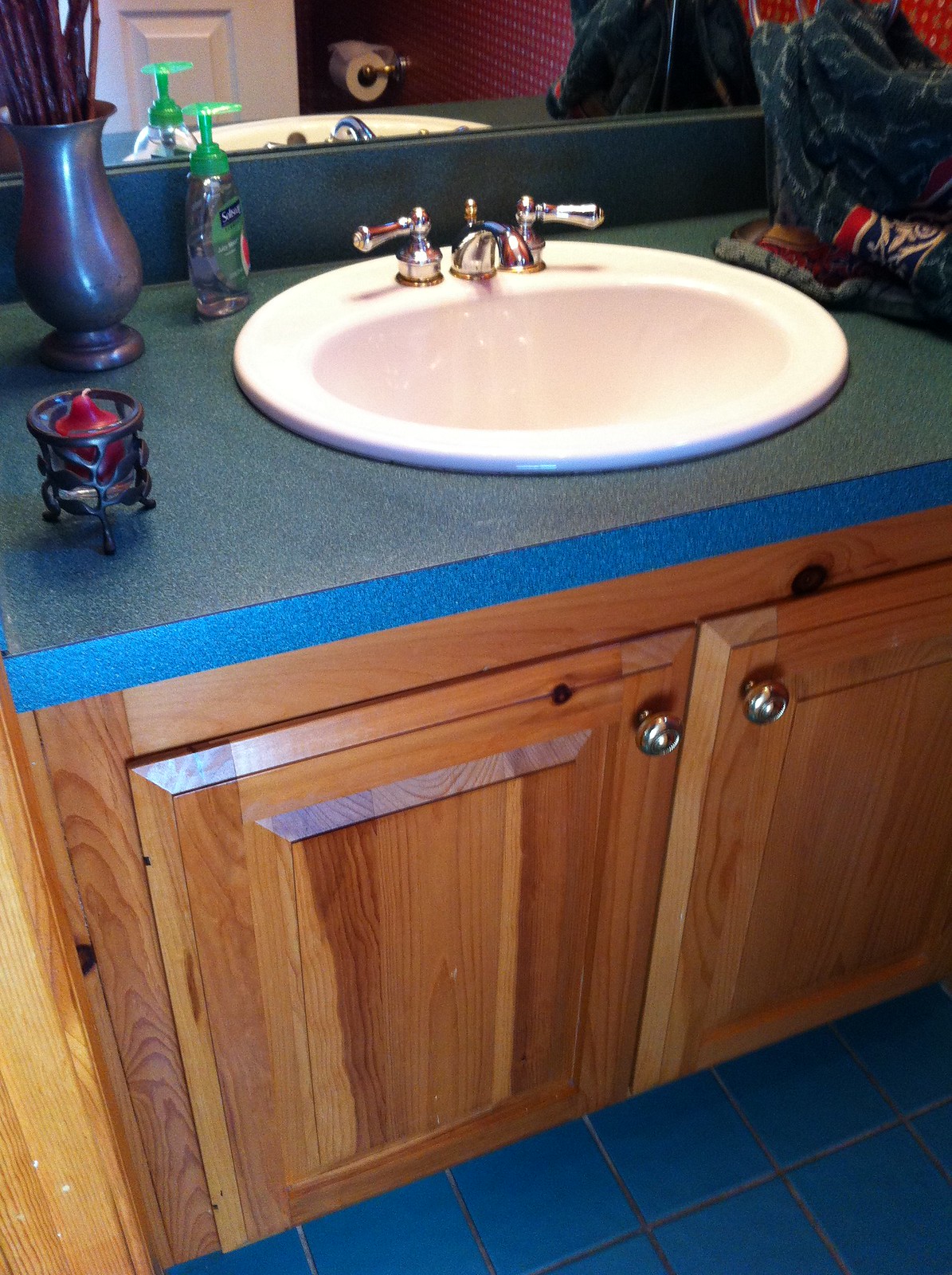The image showcases a compact, well-appointed bathroom. The floor is adorned with blue tiles, creating a cool, serene foundation for the space. A light brown wooden cabinet with elegant silver knobs stands out, topped with a striking blue countertop. Situated on the countertop is a pristine, white, oval-shaped sink, complemented by its silver handles and spout. Adding a touch of warmth and ambiance, a black candle holder containing a red candle is placed next to the sink, alongside a stylish blackish-gray flower vase with long brown stems. 

A large mirror behind the sink reflects a white door, extending the sense of space, and the reflection also captures hints of the sink area. The backdrop features a bold, red-tiled wall, adding a vibrant splash of color to the room. A roll of toilet tissue is easily accessible, while a cloth, patterned in blue, red, and white, rests nonchalantly at the end of the cabinet, adding a casual touch to the neatly arranged bathroom.